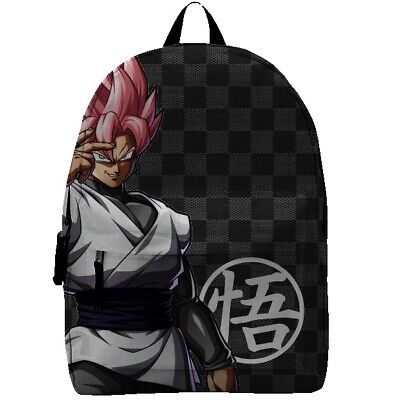This high-quality image features a basic yet striking anime-themed backpack, set against a solid white background. The backpack itself stands upright, showcasing its black and dark gray checkered pattern, which resembles a classic checkerboard. It includes a single zippered pocket in the center front. A thin, black fabric strap is visible at the top.

The focal point of the design is an anime character positioned on the left side of the backpack. This character sports spiky pink hair and menacing eyes, dressed in a white karate uniform with a black belt. Underneath the uniform, he wears a long-sleeved gray shirt and matching gray pants. His skin is light in color, and he points a finger outward. Complementing the character, a large white circle with Japanese characters is located on the lower right-hand side of the backpack.

This detailed and visually appealing book bag seems tailored for anime enthusiasts, resembling products typically found at specialty stores like Hot Topic.